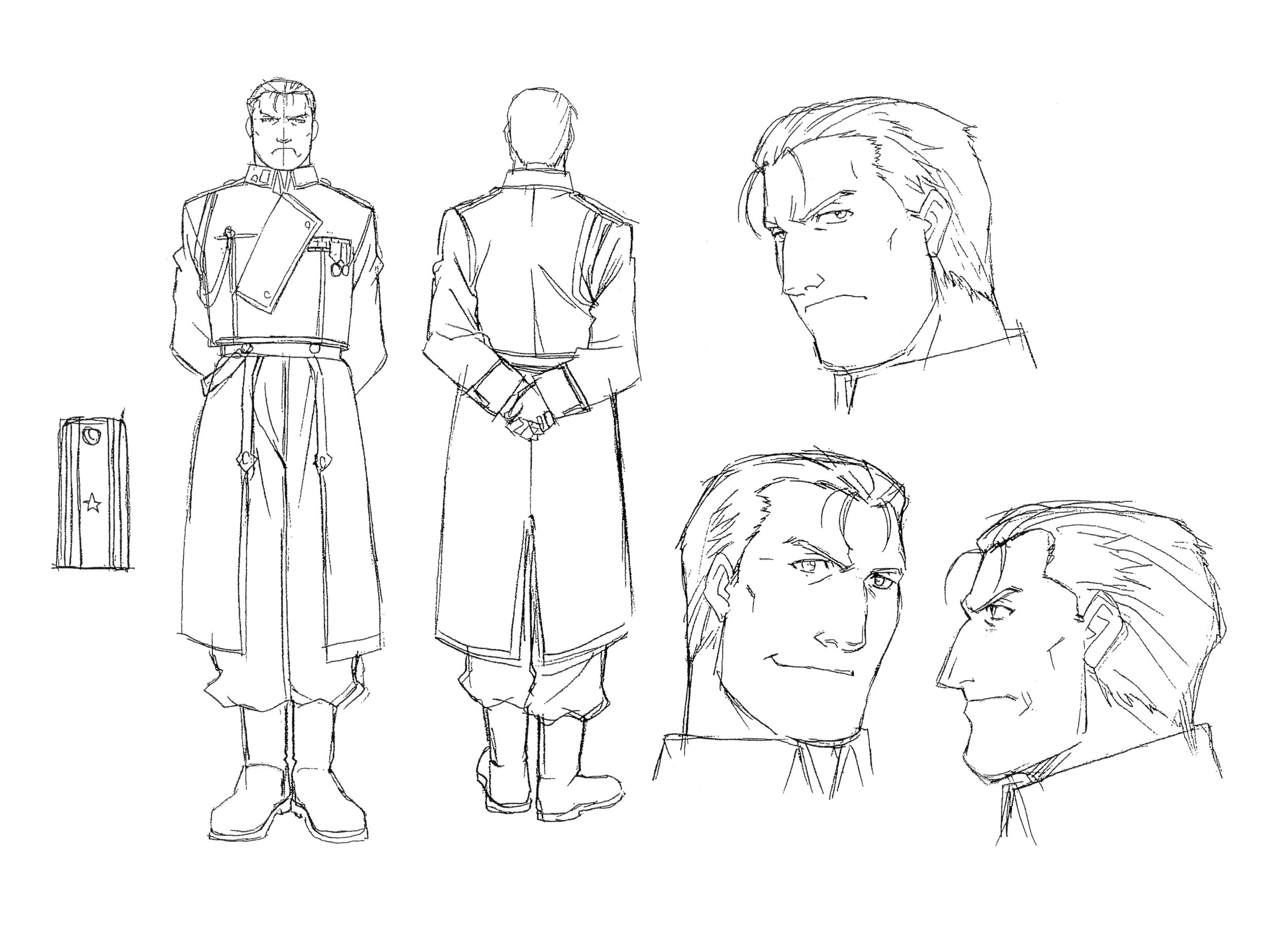This black-and-white comic book-style illustration, oriented in landscape, showcases multiple detailed views of a character dressed in a long duster coat reminiscent of a general's or officer's uniform. The character, a male with short hair that falls slightly on his forehead, is depicted in both front and back full-body sketches. The front view shows him standing with arms folded behind him, wearing heavy boots, tucked-in knickers, and a coat with an epaulette on the left shoulder adorned with a star. A chain stretches over his right arm and shoulder. The back view mirrors his stance with hands folded and similarly detailed attire. 

To the left of the character sketches, there is a vertical rectangle highlighting a specific garment detail, while the right side of the illustration is dominated by three headshots of the character. The uppermost headshot captures him in profile with an angry expression looking upward towards the viewer. Below, two faces are displayed: the left features a half-smile looking up, while the right presents a neutral expression gazing leftward. The intricate black-and-white line art and the various expressions provide a comprehensive visual character study.